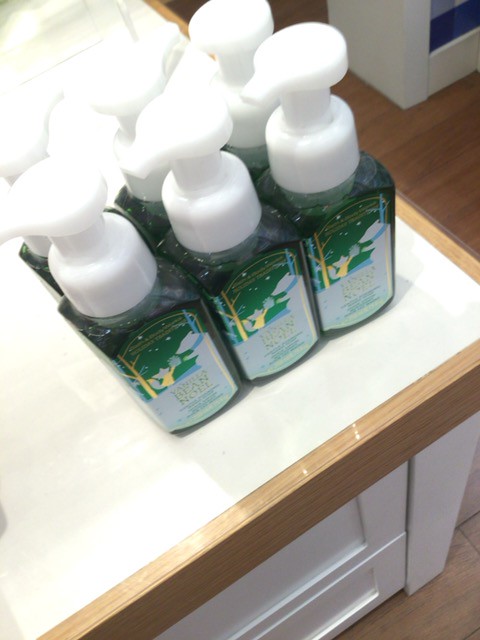This photograph features six rectangular soap bottles, each filled with green liquid soap and equipped with large white plastic pump-style caps. The bottles, likely from Bath and Body Works, display festive labels predominantly in green with touches of gold and white. These labels depict a charming winter scene in which a fox or squirrel hands a present to a polar bear, accompanied by the gold-printed text "Vanilla Bean Noel," indicating the soap's scent. The bottles are neatly lined up on a glossy white countertop, which is accented by a light blonde wood border. Below the countertop, the cabinets are painted white, and the floor is a light brown wood, suggesting the setting might be a brightly lit bathroom.